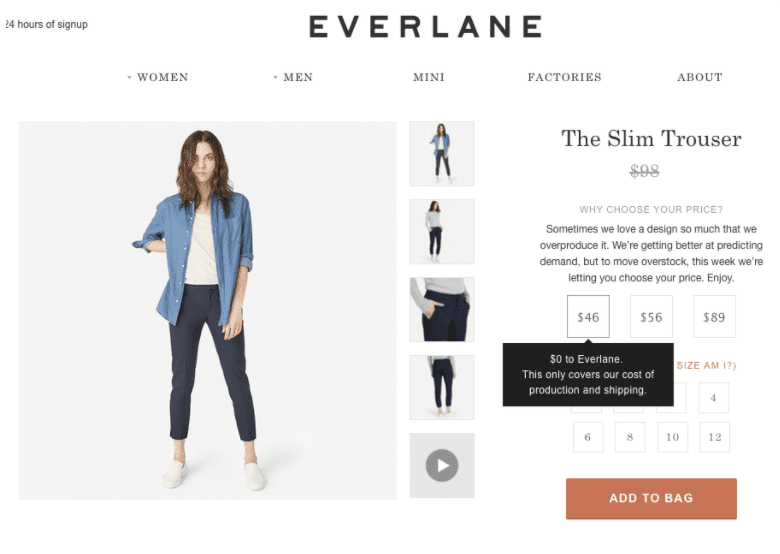The image showcases the Everlane brand prominently at the top. On the left side, under the header "24 Hours of Sign Up," are category links including "Women," "Men," "Factories," and "About." The central portion features a woman wearing an unbuttoned blue denim shirt over a white top, paired with dark blue slim trousers and white slip-on shoes, all set against a white background. To the right of this main image, there are four additional images highlighting different angles of the outfit, along with a play button on the last one, indicating a video of the slim trousers.

Adjacent to the images is a promotional section for the slim trousers. Originally priced at $98, the text "Why Choose Your Price" explains Everlane's overproduction situation and offers three selectable prices: $46, $56, and $89. Below the $46 option, it states that this amount only covers the cost of production and shipping ("$0 to Everlane"). Further down, sizes available for the trousers are listed: 4, 6, 8, 10, and 12. At the bottom, there is a dark red rectangle with "Add to Bag" written in white, signaling the option to purchase the item.